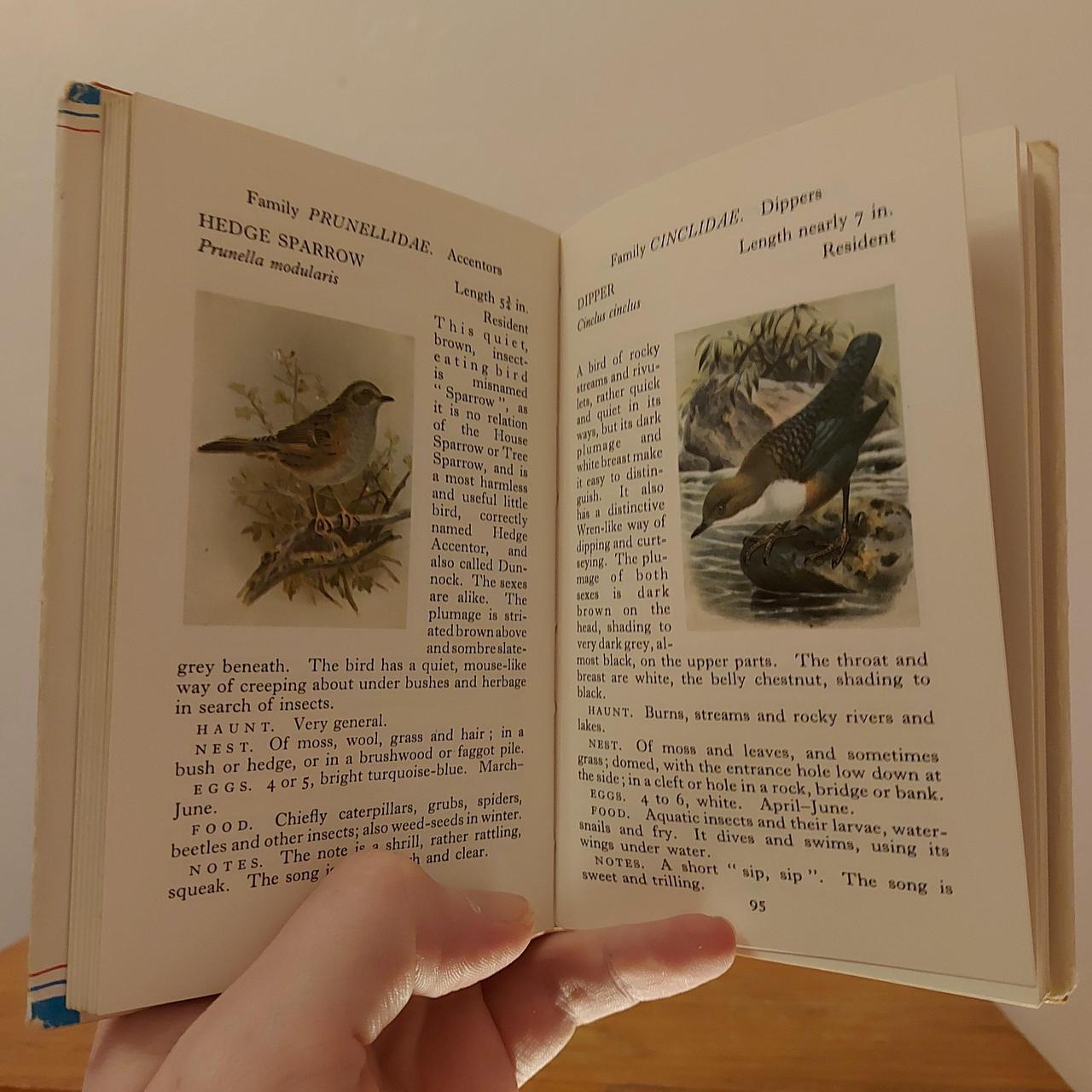The photograph depicts a man's hand holding a worn, old book open at about a 90-degree angle. The book, likely about birds, is opened to pages 94 and 95, which describe the hedge sparrow and the dipper. The page on the right is slightly creased and partially turned. The book’s edges are visibly worn, revealing hints of blue, and its paper cover shows signs of age. On the left page, the hedge sparrow is illustrated standing on twigs amidst greenery, with accompanying text describing the bird, identified under the family "Prunellidae." The right page features a larger bird, identified as a dipper, standing on a rock within a moving river, with a green body, white chest, and a brown head, neck, and part of its back. The background includes a brown wooden floor and a tan, off-white wall.